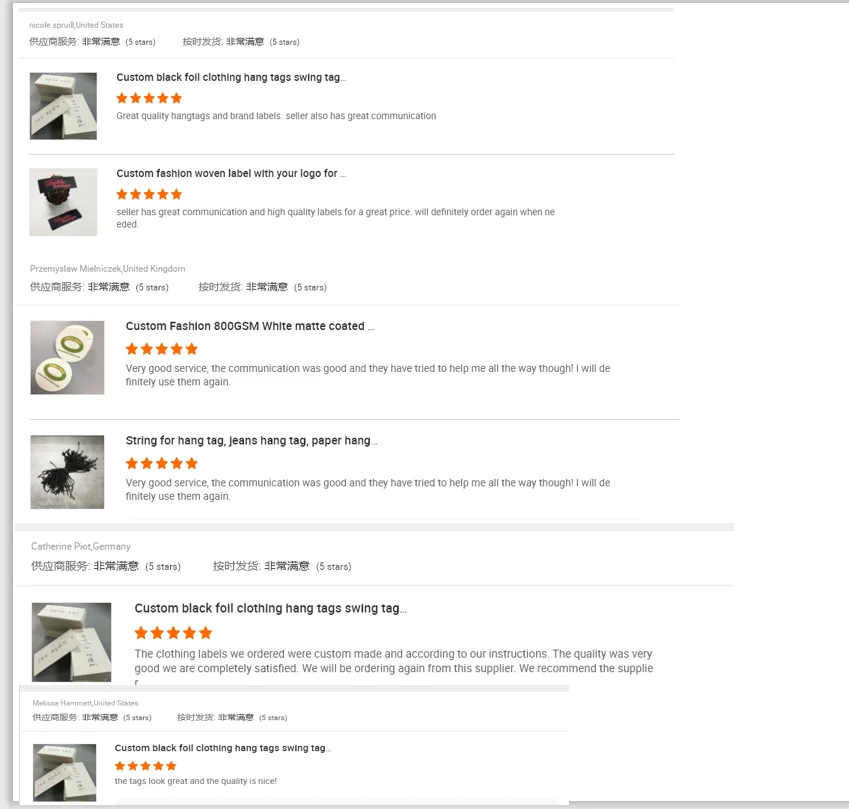Screenshot of an e-commerce website displaying a list of custom clothing store supplies. The first item on the list is "Custom Black Foil Clothing Hang Tags," followed by "Custom Fashion Woven Label with Your Logo." Another entry, partially visible, mentions "Custom Fashion 800 White Matte Coated" items. These products seem specifically tailored for clothing store owners who need custom tags and labels for their merchandise. The website is adorned with Asian characters, possibly Japanese, indicating it might be an international platform. The site also features some subsections: the first two items are listed as being from the United States by someone named Nicole, while the last two items are from Germany, associated with someone named Catherine. Overall, the layout appears somewhat complex and may be challenging to navigate.